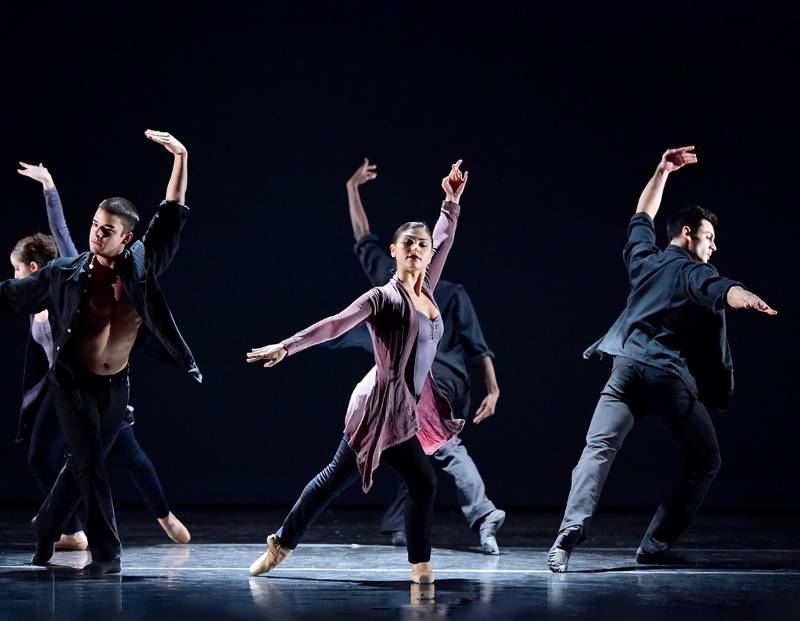The photograph captures a compelling scene of ballet dancers performing on a stage enveloped in a dark, possibly navy blue background, with a spotlight illuminating their precise movements. The floor of the stage appears smooth and reflective, creating a mirrored effect that adds depth to the image. Positioned prominently in the center, five dancers — three men and two women — each grace the floor in a similar ballet pose. Their stance reveals one hand raised above their heads and the other extended parallel to their bodies, with one knee bent and the other leg stretched back, toes pointed and touching the stage.

All dancers are clad in modern, casual attire that deviates from traditional ballet costumes. The men wear black, button-down shirts open at the front along with black pants, while the women sport tights and loose, open cardigans over their tops. The central female dancer, who stands out vividly, has medium brown skin, a light purple blouse, a blue shirt, black pants, and beige ballet slippers. Her brown hair is styled in a bun, as is the other woman's, who has lighter skin and is partially obscured. The men share a uniform look with short black hair and medium to light skin tones. Together, the dancers create a harmonious and modern visual symphony that is both captivating and elegantly understated.